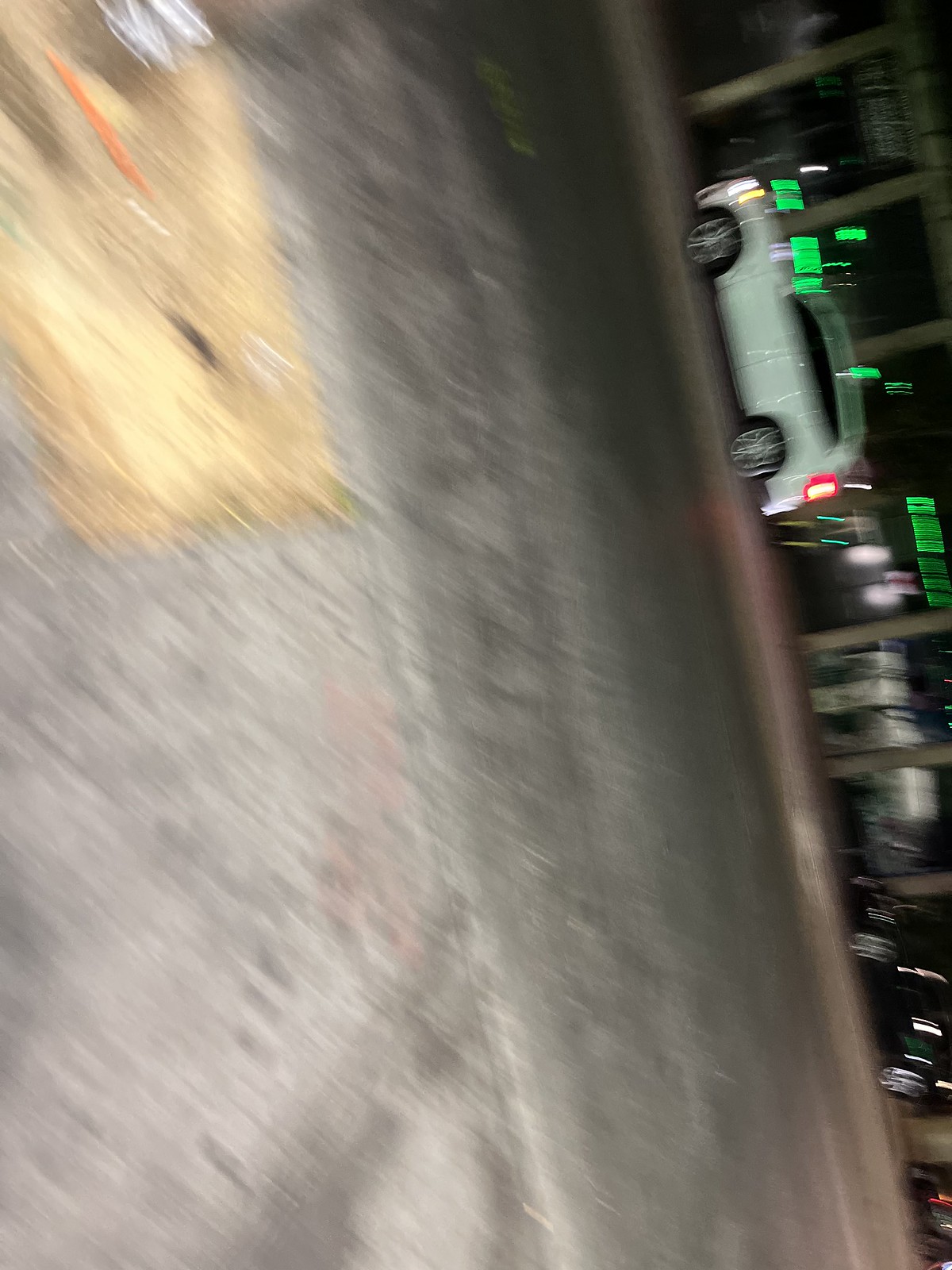An outdoor nighttime scene featuring a street with an asphalt surface tinged with a brown hue. In the top left corner, a square yellow element stands out distinctly. In the distant background, a white car is framed against a backdrop of numerous light poles that flood the area with bright illumination. A well-lit curb, glowing with a stark white light, can be seen to the left. The car in the far end has its taillight glowing, adding a touch of red to the scene. Reflective windows are visible in the background, mirroring the intense lighting. The entire composition appears to be taken on a random street, captured under the stark, artificial light of the camera's flash.